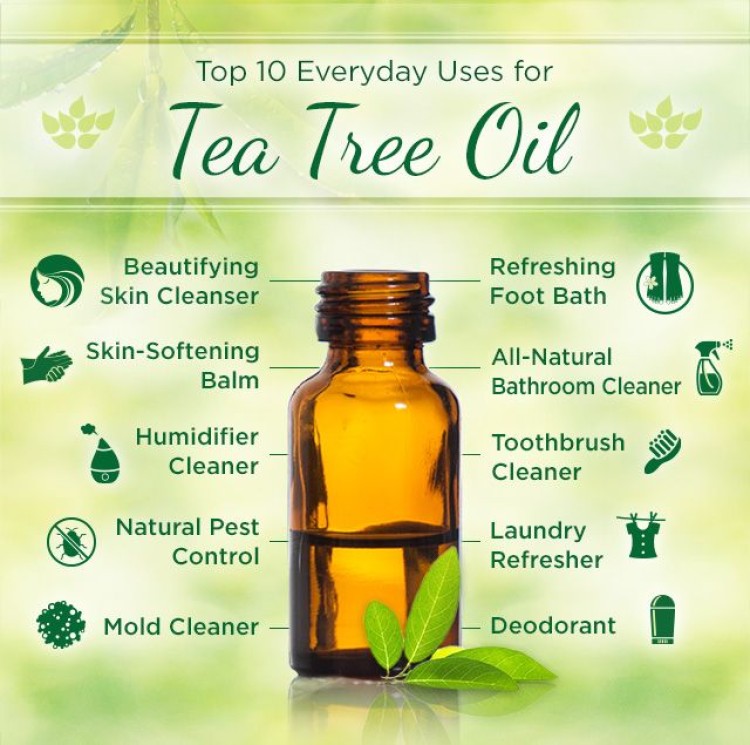This image serves as an educational resource showcasing the versatile uses of tea tree oil. Set against a light green background with a darker green banner at the top, the text boldly reads, "Top 10 Everyday Uses for Tea Tree Oil." A brown, amber bottle—approximately one-third full of tea tree oil—is central to the design, accompanied by decorative tea tree leaves at its base. The backdrop features a soft, faded image of green leaves, enhancing the natural theme.

On the left-hand side, the benefits listed are: Beautifying Skin Cleanser, Skin Softening Balm, Humidifier Cleaner, Natural Pest Control, and Mold Cleaner. On the right-hand side, the uses are: Refreshing Foot Balm, All Natural Bathroom Cleaner, Toothbrush Cleaner, Laundry Refresher, and Deodorant. Each benefit is depicted with a corresponding small emoji, adding a visual representation. This detailed visual sheet educates viewers on the everyday applications of tea tree oil in a visually appealing and organized manner.